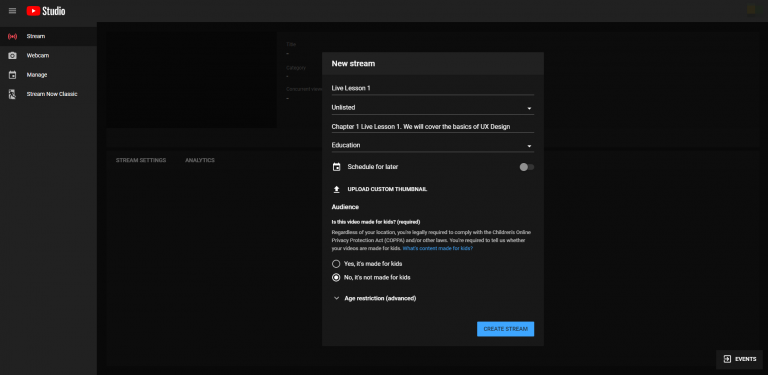Here is a comprehensive and detailed caption for the described image:

"This is a screenshot of YouTube Studio, showcasing the interface for scheduling and managing live streams. The background predominantly features a black color with a very dark gray strip along the top edge and left-hand side. At the top edge, three key icons are displayed: a three-line horizontal icon for additional options, the red YouTube Play button, and the word 'Studio' in white text.

On the left gray border, the options 'Stream,' 'Webcam,' and 'Manage' are visible. Adjacent to the 'Stream Now Classic' option, there's a black-bordered section containing a pop-up window. This window displays in white text: 'New Stream' and 'Live Lesson 1.' Below this is a drop-down menu indicating 'Unlisted.' Further down, it reads 'Chapter 1, Live Lesson 1' followed by a brief description: 'We will cover the basics of UX design,' accompanied by another drop-down menu labeled 'Education.'

There is a 'Schedule for Later' button, which is gray and points to the left. Following this, there's an 'Upload Custom Thumbnail' button and a section labeled 'Audience.' This section informs users about the requirement to comply with the Children’s Online Privacy Protection Act and other relevant laws regarding whether the video is made for kids. The options provided are 'Yes, it’s made for kids,' or 'No, it’s not made for kids,' with the 'No' option currently selected. Finally, at the bottom right, a blue 'Create Stream' button is present."